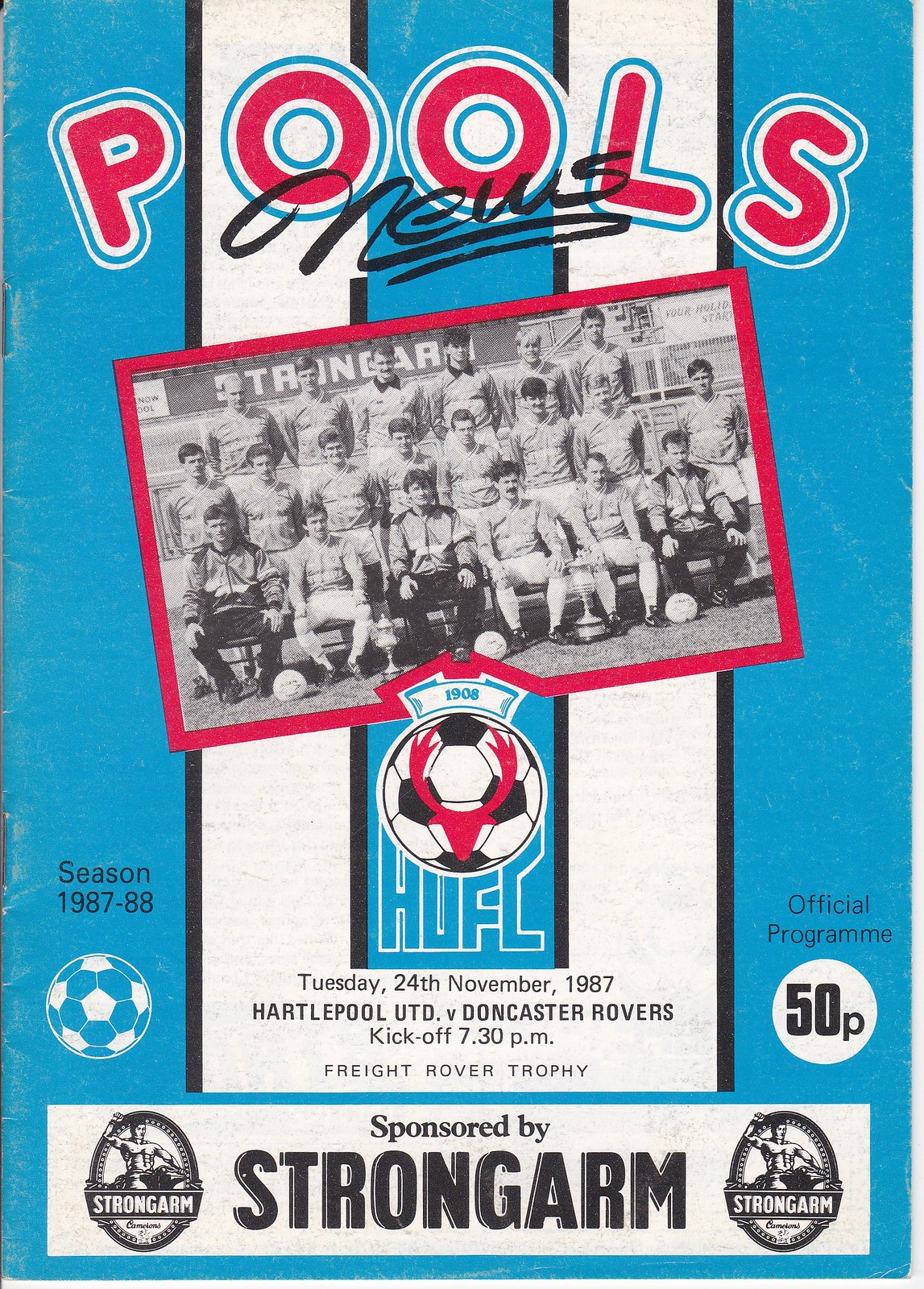The image is a tall, rectangular sports program with a bright blue background punctuated by white smudges. Dominating the top portion, bold red letters outlined in white and blue announce "POOLS" with "NEWS" in black script beneath. Centrally featured is a vintage black-and-white photograph of a soccer team posed in three rows, the front row seated while the two behind stand. This photo is framed by a red border. Below this, a white soccer ball sports a striking red stag caricature at its center and the letters "H-U-F-C". An informational section beneath reads, "Tuesday, 24 November, 1987, Hartlepool UTD vs. Doncaster Rovers, kickoff 7:30 PM," indicating the event is part of the Freight Rover Trophy. To the left is a depiction of a blue and white soccer ball with the notation “Season 1987-88,” and to the right, a white circle declares this as the “official program” priced at 50p. At the page's bottom, a white rectangle boldly states "sponsored by STRONGARM," flanked by the Strongarm logo.